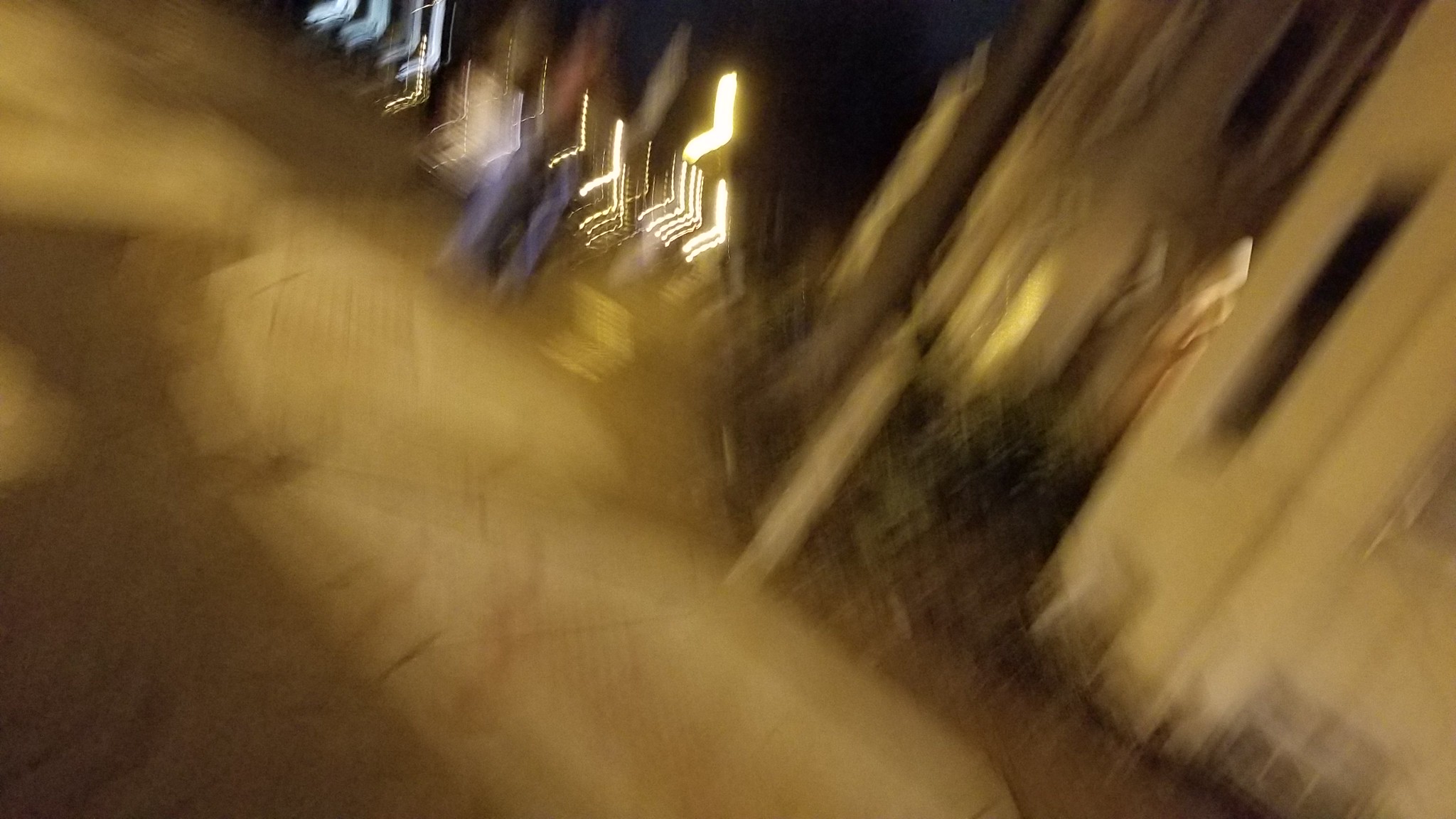The image depicts a very blurry street corner scene at night with a yellowish tint. The left side of the photo shows a dark brown triangular shape, possibly a structure, with lighter brown swirls on the ground, suggesting the sidewalk or road. To the right, the edge of a beige-colored building with doorways and windows is visible. There are bright street lights in the top left corner, likely from vehicles or nearby buildings, illuminating the scene. Near the building, street signs with blue and white arrows indicate a turn in the road. A faint outline of a figure in blue pants can be discerned in the distance. The overall scene is characterized by its poor clarity, but the essential elements of buildings, street lights, and directional signs are distinguishable.